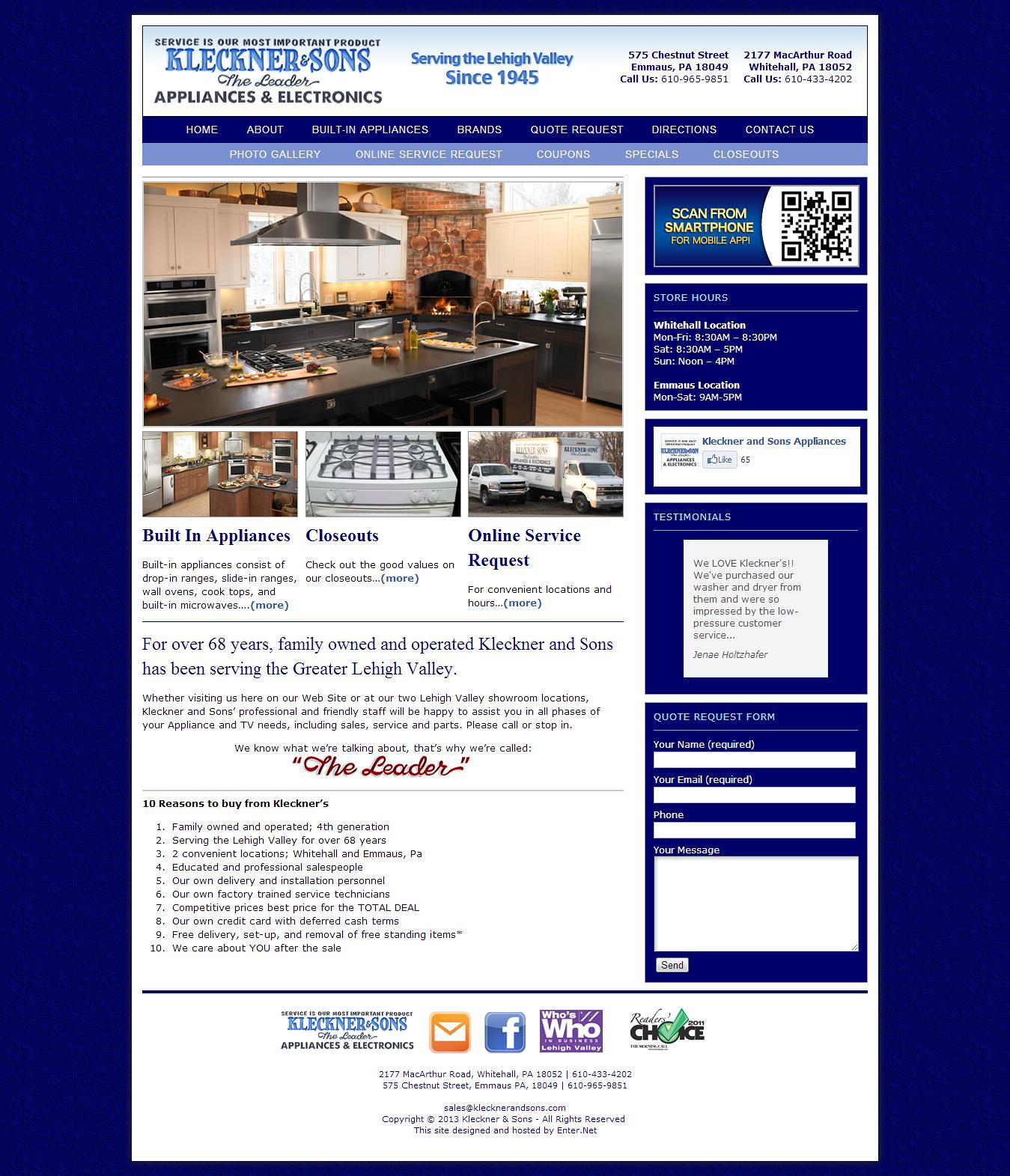The pamphlet is a detailed advertisement for Kleckner & Sons, a family-owned and operated business serving the greater Lehigh Valley for over 68 years. At the upper left corner, the pamphlet prominently features the heading, "Kleckner & Sons: The Leader in Appliances and Electronics." Below this, a large, captivating landscape image showcases a modern kitchen complete with a countertop, chimney, built-in ovens, gas stoves, refrigerator, kitchen platform, fireplace, windows, faucets, and utensils. 

Adjacent to this image, the pamphlet is adorned with additional photographs labeled "Built-in Appliances," "Closeouts," and "Online Service Requests." The built-in appliances image depicts various high-end kitchen installations, including drop-in ranges, wall ovens, and cooktops. The closeouts section highlights significant savings on appliance closeouts, while the online service requests area facilitates convenient service bookings.

In the middle of the pamphlet, a bold proclamation states, "For over 68 years, family-owned and operated, Kleckner & Sons has been serving the greater Lehigh Valley." This section emphasizes the store’s longevity and commitment to customer service, backed by the tagline "The Leader," written in prominent red text.

The top right corner lists the company’s two store locations and their respective addresses: 575 Chestnut Street, Emmaus, PA, 18049, and 2177 MacArthur Road, Whitehall, PA, 18052, along with contact numbers for each location. Additionally, it details store hours for both locations, incorporates a QR code to download their mobile app, and features a Facebook logo with user testimonials and engagement buttons.

The bottom section of the pamphlet provides ten compelling reasons to shop at Kleckner & Sons, emphasizing their family ownership, long-standing service, convenient locations, professional staff, proprietary credit options, and post-sale care. It also includes a section for a quote request form, complete with fields for name, email, phone, and message.

Overall, the pamphlet meticulously illustrates Kleckner & Sons' dedication to superior service and quality products, enhanced by professional design elements and comprehensive customer-centric information.